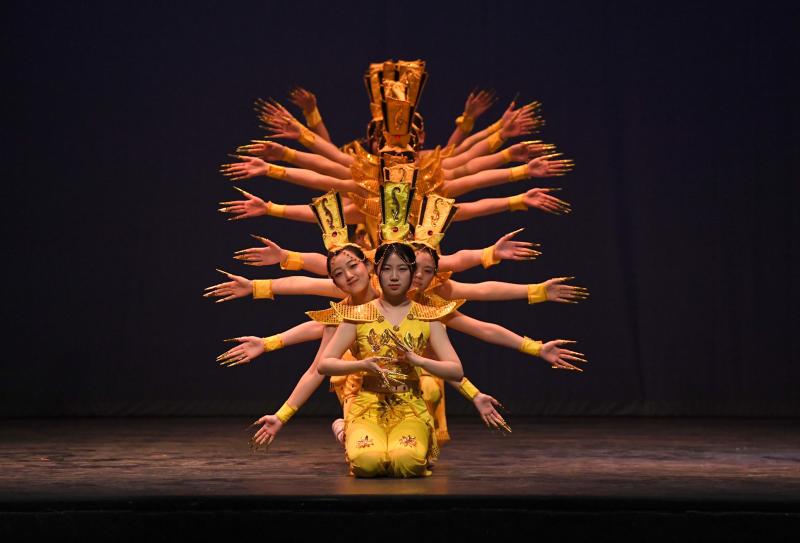This vibrant square photo, captured indoors under artificial lighting, showcases an intricate performance on a polished brown wooden stage framed by black curtains with a subtle trim at the bottom. Central to the composition is a young Asian woman, kneeling gracefully at the forefront, adorned in a striking yellow outfit complete with a matching headpiece, evocative of traditional Chinese attire. Her arms are elegantly outstretched, creating a mesmerizing illusion as numerous pairs of arms, uniformly clad in yellow wristbands, extend from behind her in perfect synchronization. The arrangement of these arms, belonging to other similarly dressed performers, radiates outward, mimicking the image of a sunburst or the multi-armed depiction of a deity, hinting at an artistic dance technique. This tableau, with each element meticulously positioned, prepares the audience for an enchanting traditional dance performance, capturing a moment of poised anticipation and intricate beauty.